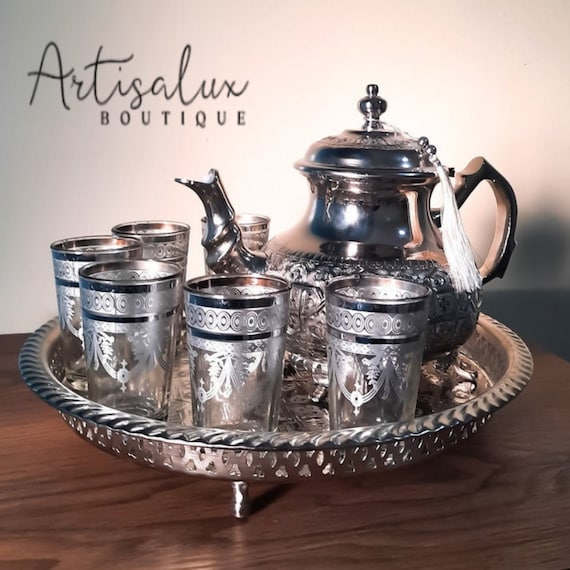This indoor, perfectly square photograph features an antique-style tea set elegantly presented on a dark, brown wooden table against a white wall. In the top left corner, dark gray text reads "Artesilux Boutique," with "Artesilux" written in cursive and "Boutique" in a standard font. The background fades from the white wall to a pinkish tone and then to gray. Central to the image is a silver plate resting on thin, elevated metal legs. Ornately designed silver and black glasses form a U-shape around an exquisite silver tea kettle, which is adorned with a white tassel on its top. The glasses are clear towards their bottoms and feature intricate designs near their tops, including silver patterns and white etchings. The tea kettle, positioned on the right side of the silver plate, is an ornate metal piece with a handle, a top, and a spout, contributing to the overall sophisticated arrangement.